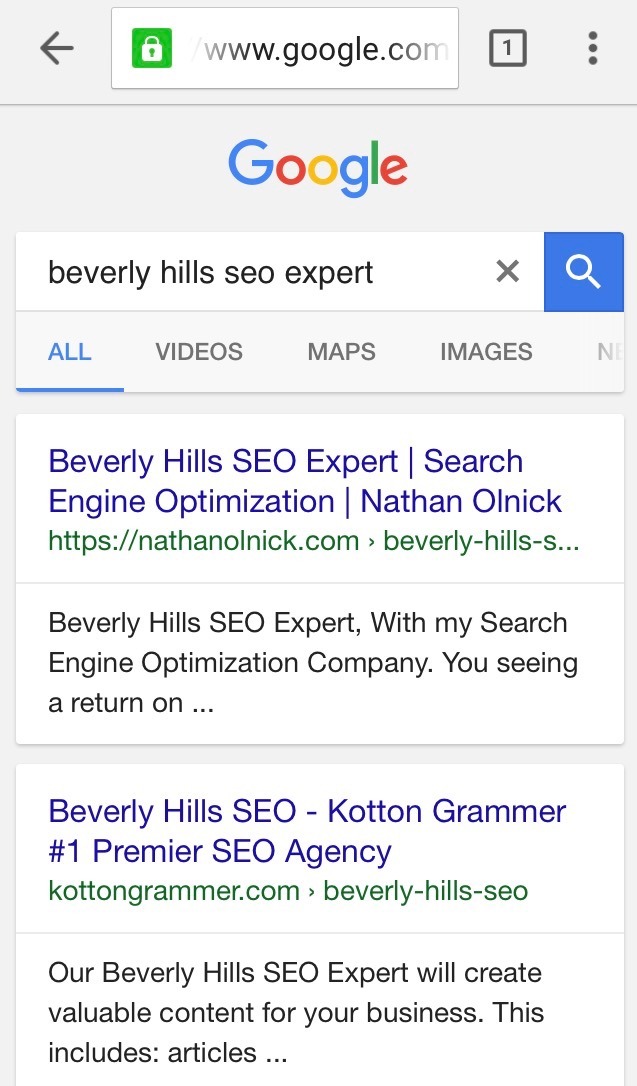The image depicts a Google search result page. At the top of the page is the familiar Google logo with the search query "Beverly Hills SEO expert" entered into the search bar. The search results are displayed under the "All" tab, indicating that the user is viewing a comprehensive list of results. 

The first search result is highlighted in blue text reading "Beverly Hills SEO Expert - Search Engine Optimization by Nathan Olnick," with the URL "nathanolnick.com" shown in green text beneath it. This result includes a brief snippet that begins with the phrase, "Beverly Hills SEO expert with my search engine optimization company you seeing a return on..."

The second result also appears in blue text and reads "Beverly Hills SEO - Cotton Grammar #1 Premier SEO Agency." Similar to the first result, its URL "cottongrammar.com" is displayed in green text beneath the title. The snippet provided for this link starts with, "Our Beverly Hills SEO expert will create valuable for your business this includes articles..."